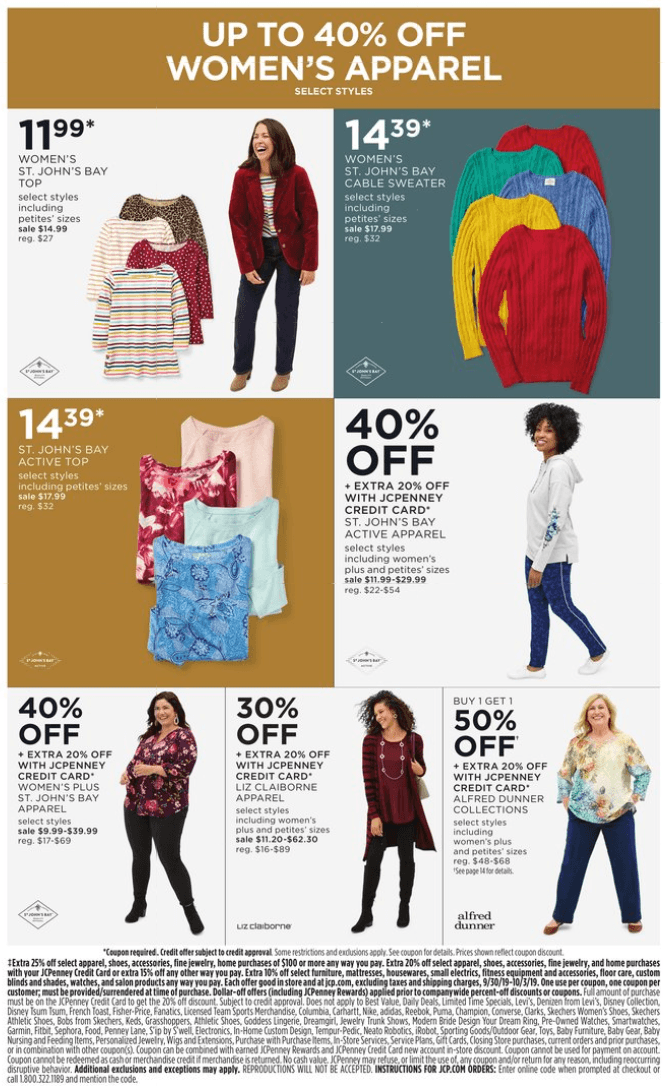This vibrant and cheerful web advertisement exudes the classic feel of Sunday newspaper print ads, offering significant discounts on women's apparel. Dominating the page is a headline announcing "Up to 40% Off Women's Apparel," and showcasing seven distinct promotions with discounts of up to 50% off on various stylish and affordable clothing. The paramount focus is on the extensive sale, although the retailer’s identity, revealed only in fine print, is JCPenney.

In the upper left corner, the mention of "St. John's Bay" subtly ties the ad to JCPenney, confirmed by the highlighted offer of "40% off when you open a JCPenney credit card." The ad's design is enlivened by bright, cheerful colors and images of smiling women modeling the featured clothing. The diversity of the models stands out, with several plus-size women included, highlighting the retailer's inclusive approach.

Among the featured items, there are stylish tops, cozy long-sleeved tops, and snug sweaters. The athletic section showcases a model in a comfortable hoodie and exercise pants, promoting "40% off active apparel." Other remarkable discounts include "30% off Liz Claiborne products" and "50% off Alfred Dunner collections," catering to a range of fashion preferences. The detailed fine print at the bottom provides the essential terms and conditions of the discounts.